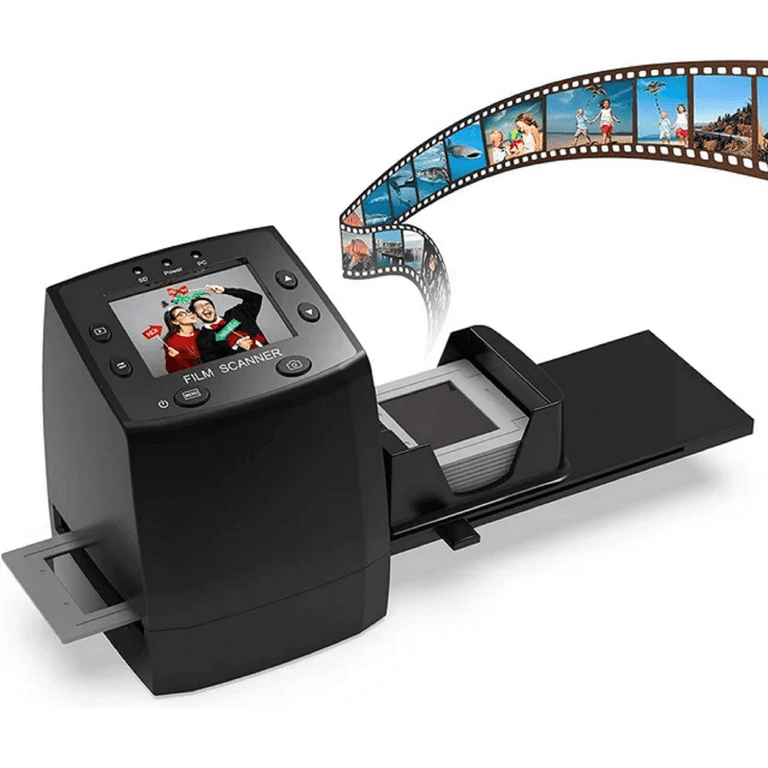The image features a black, tall, square-shaped device prominently labeled as a "film scanner" at the top. A digital display above this label showcases a celebratory scene with a man and a woman dressed in festive apparel, possibly indicating Christmas or New Year's, holding picture props like a red arrow. The device has a central, large, rectangular plastic panel that appears to hold photographic slides or film negatives. Running through the scanner is a film strip, which emerges from the bottom, indicating the scanner's purpose of digitizing old film rolls. The display additionally supports arrow buttons on both sides, along with a power and a camera button, highlighting its functional versatility. The overall theme of the displayed images suggests an aquatic, beach-like setting, likely to showcase various moments captured on film. This comprehensive depiction suggests that the film scanner is designed to convert traditional film into digital format, allowing further use on computers or smartphones.